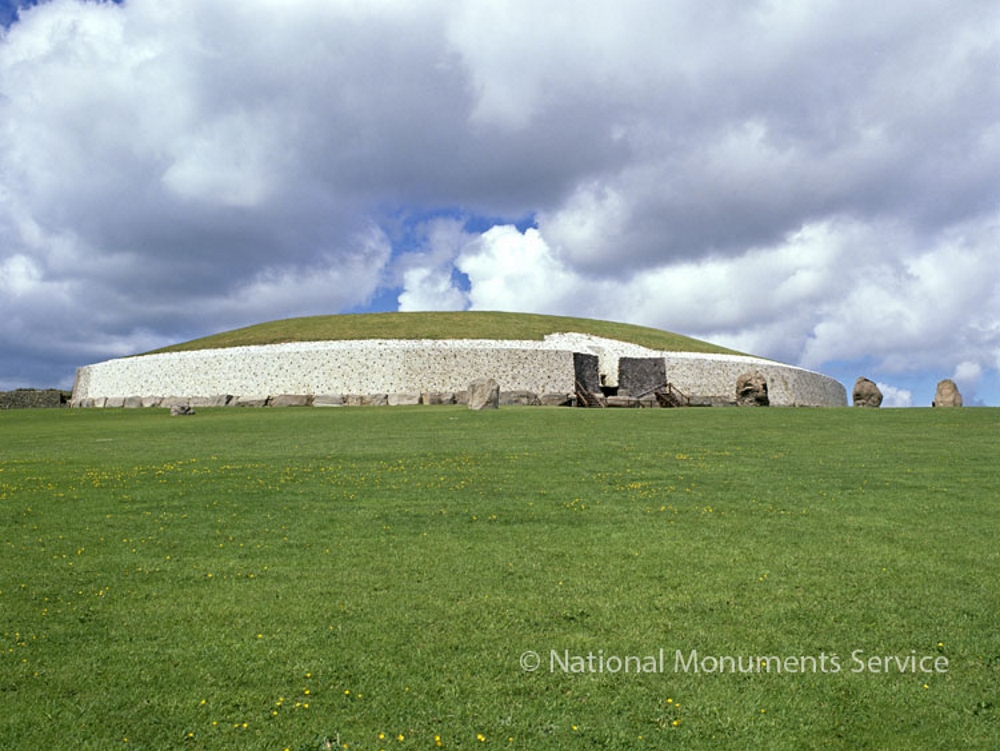This is a photograph of a national monument, specifically a large, circular concrete structure with a white, oval shape and a ceiling covered in grass. The monument is set in the middle of a beautifully manicured field of vibrant green grass dotted with small yellow wildflowers. Surrounding the structure are numerous large boulders arranged in an intentional pattern, with four of these standing upright outside the main building. The image captures a dramatic sky filled with dark, heavy clouds allowing rays of sunlight to peek through, creating a stunning contrast against the blue backdrop. The photo, taken from ground level as if the viewer is sitting on the grass, highlights the imposing presence of the structure, which appears older and might be accessible to walk through, featuring an opening with stairs. This iconic image, complete with a copyright from the National Monuments Service, would be a perfect visual attraction for a website encouraging visitors to explore this historical landmark.